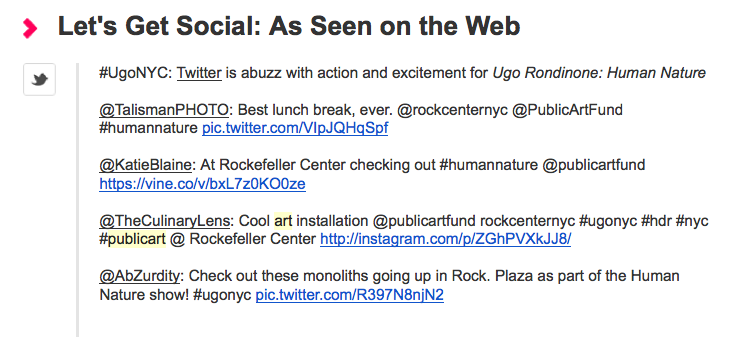Here is a cleaned-up and detailed descriptive caption based on the image and voice description provided:

---

At the top of the image is a pink, arrowhead-like shape pointing to the right. Next to this arrowhead, in bold black text, is the phrase "Let's get social..." followed by, "As seen on the web." Directly below this text, there is a blue Twitter symbol. A thin, vertical green line separates the Twitter symbol from more text. On the other side of the green line, in black text, it reads: "#UGONYC... It's abuzz with the action and excitement for 'You Go Run' by Ron Dinone... Human Nature."

Following this, there is a phrase and tag sequence: "@telusmenphotos... Best lunch break ever, at Rockefeller Center NYC, @PublicArtFund, #HumanNature." Below, a link directs viewers to a Vine video: "@KatieBlaine at Rockefeller Center checking out #HumanNature at @PublicArtFund." Additional space follows before the next phrase: "@culinarylands... Cool art installation at @PublicArtFund, Rockefeller Center, NYC," with hashtags: #UGONYC, #HDR, #NYC, #PublicArt. Then, an Instagram link is provided to view the image.

The final part of the caption reads: "@absurdity... Check out these monoliths going up in Rockefeller Plaza as part of the Human Nature show, #UGONYC," accompanied by a Twitter picture link.

---

This version provides a clear and organized transcription with detailed descriptions of the social media engagement referenced in the image.